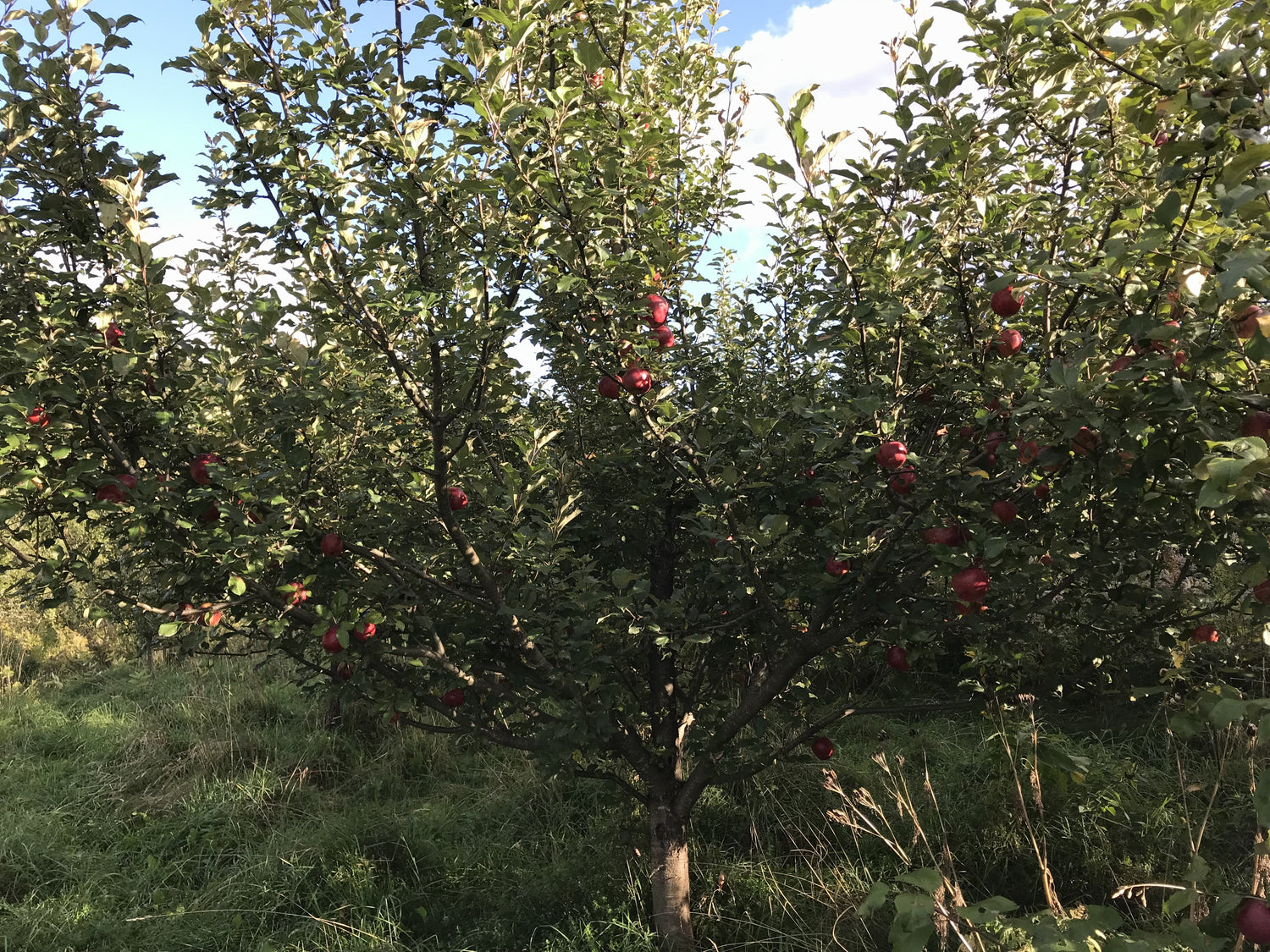The photograph captures an outdoor scene with a tree-like bush that is too short to be an actual tree. This bush has a thick brown trunk at its center, although it remains too thin to classify as a true tree. Its brown branches spread out low to the ground, laden with teardrop-shaped green leaves and adorned with small, spherical red fruit, reminiscent of apples. Multiple similar bushes flank it on both the right and left. The sky above is visible through the branches, revealing a pleasant light blue expanse dotted with white clouds, suggesting a sunny daytime setting. Below the bush, the ground is covered with clumps of tall green grass and scattered yellow weeds, contributing to the natural, serene outdoor ambiance.